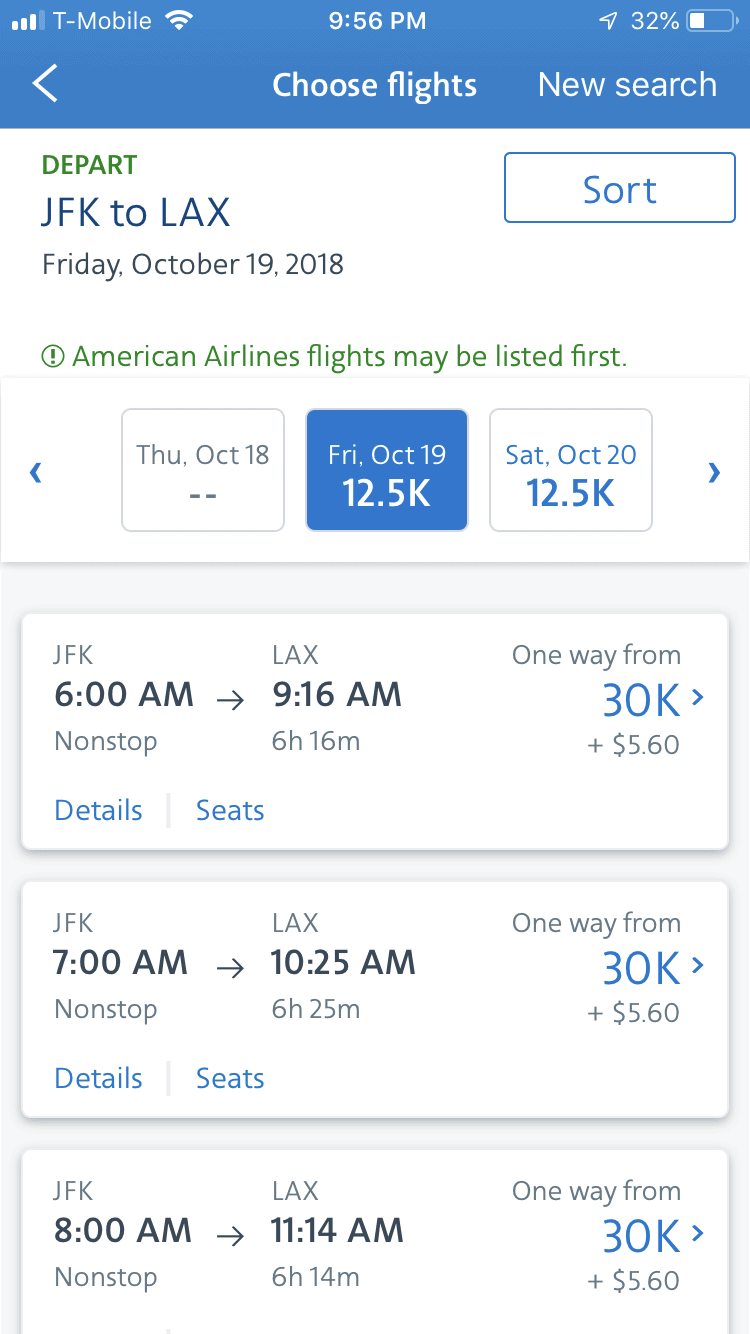This portrait mode screenshot captures a flight search interface on a mobile device. At the top, a light blue stripe spans the upper part of the screen, displaying essential device information in white: "T-Mobile" in the top left, "9:56 PM" in the center, and a battery icon indicating 32% in the top right. Below this strip, there are a few navigational buttons: a white back button on the left, and "Choose Flights" and "New Search" to the right.

The main content is organized in a vertical column with a white background. At the top left, the text "Depart" is highlighted in green. Below this, the departure and destination airports "JFK to LAX" are displayed in blue, along with the travel date "Friday, October 19, 2018."

To the right, there's a "Sort" button in blue. Beneath this, a green text warns, "American Airlines flights may be listed first." There's also a scroll menu with selectable dates and prices: 
- "Thursday, October 18th" with a "Clear" button.
- "Friday, October 19th," highlighted in blue with "12.5K" (presumably reward points).
- "Saturday, October 20th," showing "12.5K" as well.

Listed flights follow:
1. Flight from JFK at 6:00 AM, arriving at LAX at 9:16 AM, marked as "Non-stop, 6 hours 16 minutes." Below, "Details" and "Seats" are available links in blue. This flight is priced at "30K points plus $5.60 USD" for a one-way ticket.
2. Another flight, departing JFK at 7:00 AM and arriving at LAX at 10:25 AM, also priced at "30K" points.
3. The last flight, leaves JFK at 8:00 AM and lands at LAX at 11:14 AM, similarly priced at "30K" points.